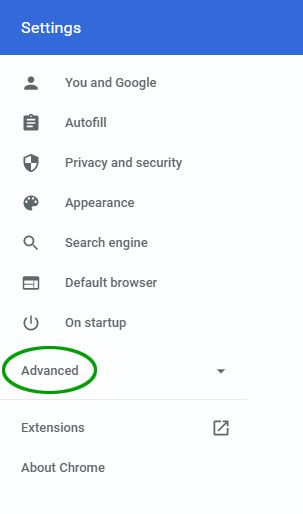The image depicts a settings page on a mobile device. At the top, there is a blue banner with the word "Settings" written in white on the left side. Below this banner, the background is entirely white. The subsequent sections are labeled in black text.

The first section, titled "You and Google," features a small, black person icon. 

The second section is "Autofill," represented by a black square containing three horizontal white lines, resembling a notepad.

Following that is the "Privacy and Security" section, indicated by an emblematic banner in a mix of black and white.

The "Appearance" section is next, denoted by an icon resembling a painter’s palette with black body and white dots.

The "Search Engine" section is represented by a black search bar icon.

For the "Default Browser" section, there is a black square with a white center, bisected both vertically and horizontally.

Next is the "On Startup" section, symbolized by a black three-quarter circle with a vertical line at the top.

On the left side, "Advanced" is outlined in a green marker, forming an oval around the word. There is a downward-pointing arrow next to it.

Below a thin gray separating line, the "Extensions" section appears, accompanied by a small black box with an arrow pointing diagonally up to the right.

Finally, under the "Extensions" section, there is "About Chrome."

Each section is distinctly marked, making the navigation intuitive and organized.